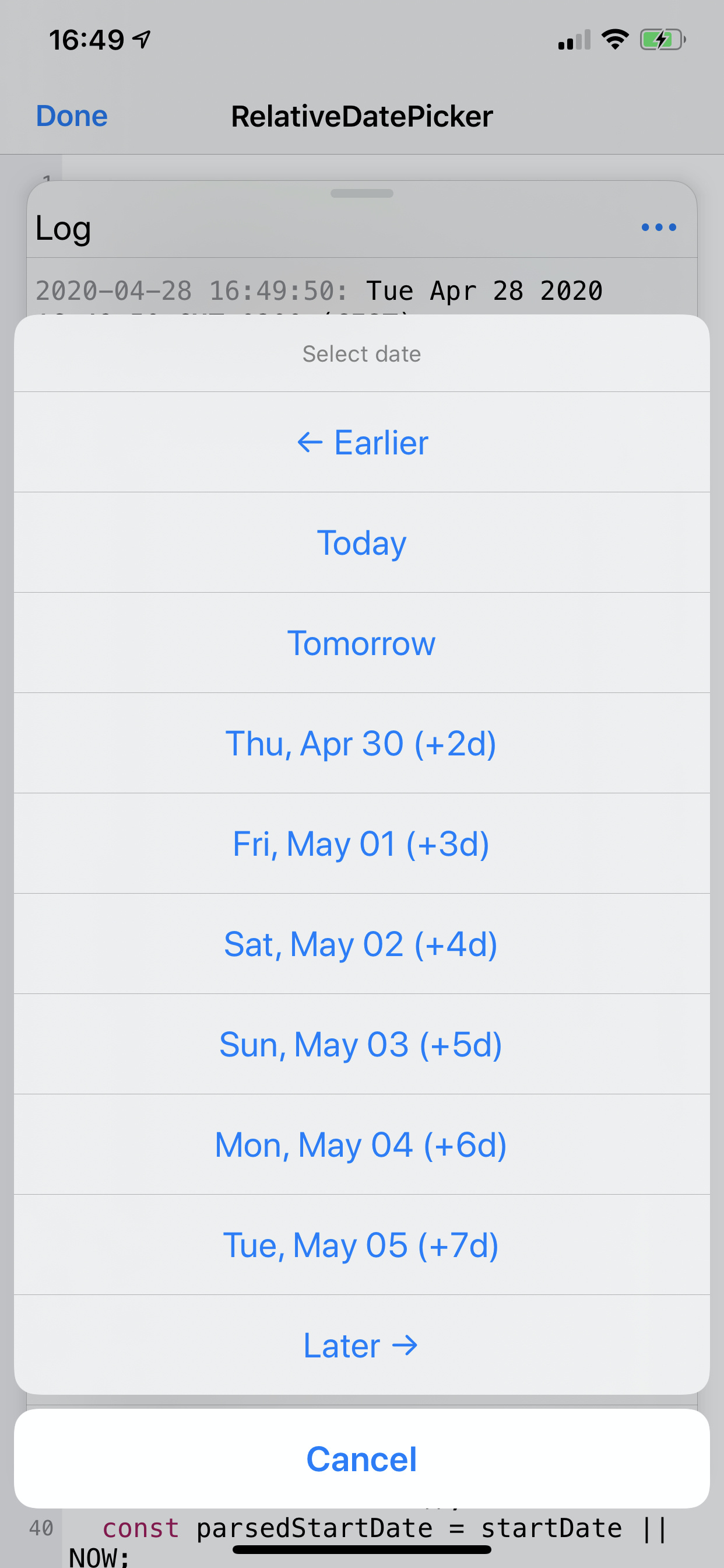The screenshot features a dark green rectangular background at the top, predominantly occupied by various interface elements. At the top left, the time "10:49" is displayed in black text. Adjacent to it are icons indicating the internet signal strength, internet connectivity, and a battery icon glowing green. 

Below the status bar, the next section of the interface is a blue button labeled "Done," and next to it, a black text reads "Relative Date Picker." Following this, there is a gray rectangular field with the word "Log" in black, alongside gray numerical values and the date "Tuesday, April 28th, 2020."

Beneath this, a prompt in gray text instructs to "Select date." This is followed by a series of options within a light gray rectangular background, each encapsulated in blue text. They read as follows from top to bottom:
- "Earlier" followed by a left-facing arrow,
- "Today,"
- "Tomorrow,"
- "Thursday, April 30th (+2 day),"
- "Friday, May 1st (+3 day),"
- "Saturday, May 2nd (+4 day),"
- "Sunday, May 3rd (+5 day),"
- "Monday, May 4th (+6 day),"
- "Tuesday, May 5th (+7 day),"
- "Later" followed by a right-facing arrow.

At the bottom of this list, a white rectangular button displays the word "Cancel." 

The remaining section of the dark green rectangle displays text in red: "c-o-n-s-t," followed by code: "parsed start date = start date." This code snippet is partially underlined by a solid black line.